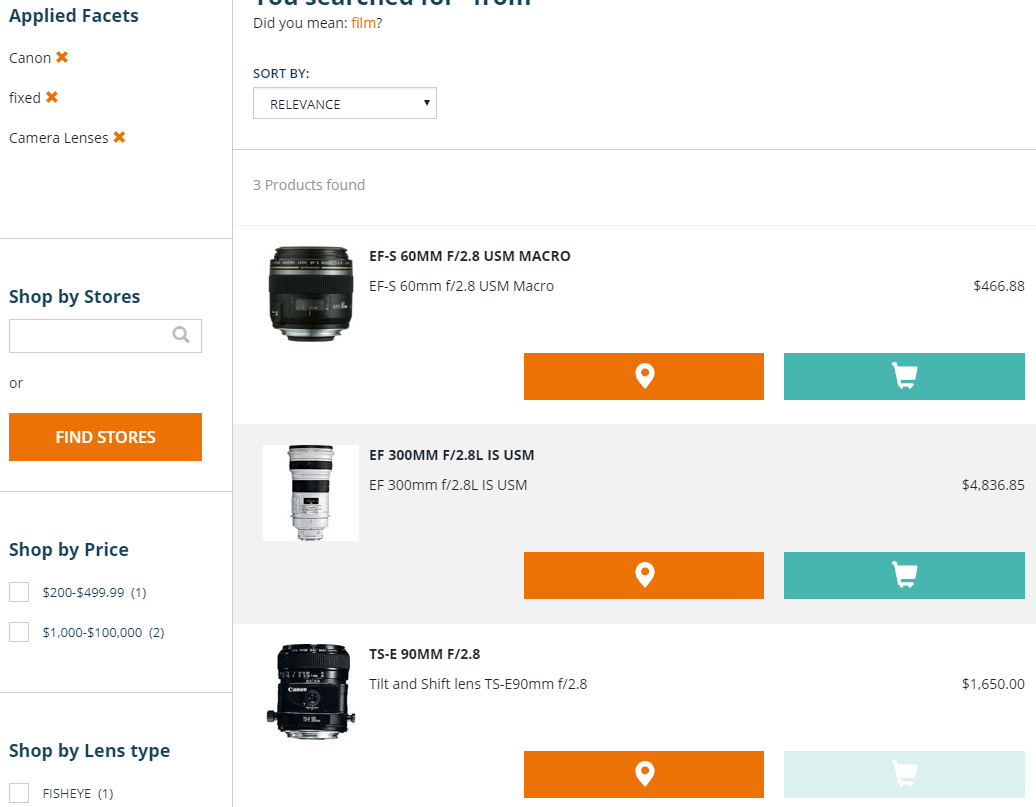The image depicts a webpage from an unidentified website, likely related to camera equipment, featuring a selection of camera lenses for sale. On the left side of the webpage, under a column titled 'Applied Facets,' there are specific search criteria listed with orange crosses allowing for deselection. These criteria include 'Canon,' 'Fixed,' and 'Camera Lenses.' Below this, a search box allows users to 'Shop by Stores,' with an option to 'Find Stores' via an orange button. Two checkboxes for 'Shop by Price' display price ranges: $200 to $499.99 and $1,000 to $100,000.

In a wider column to the right, three distinct camera lenses are showcased. The top lens is an EF-S 60mm lens, priced at $466.88, accompanied by an image of the lens on its left. To the right and below the lens description, there are icons for adding the item to a shopping cart and for locating stores. The second item listed is a long EF 300mm F2.8L lens, priced at $4,836.85, with similar accompanying icons. The final item is a TSE 90mm lens, priced at $1,650, also complete with an image and the same set of functional icons.